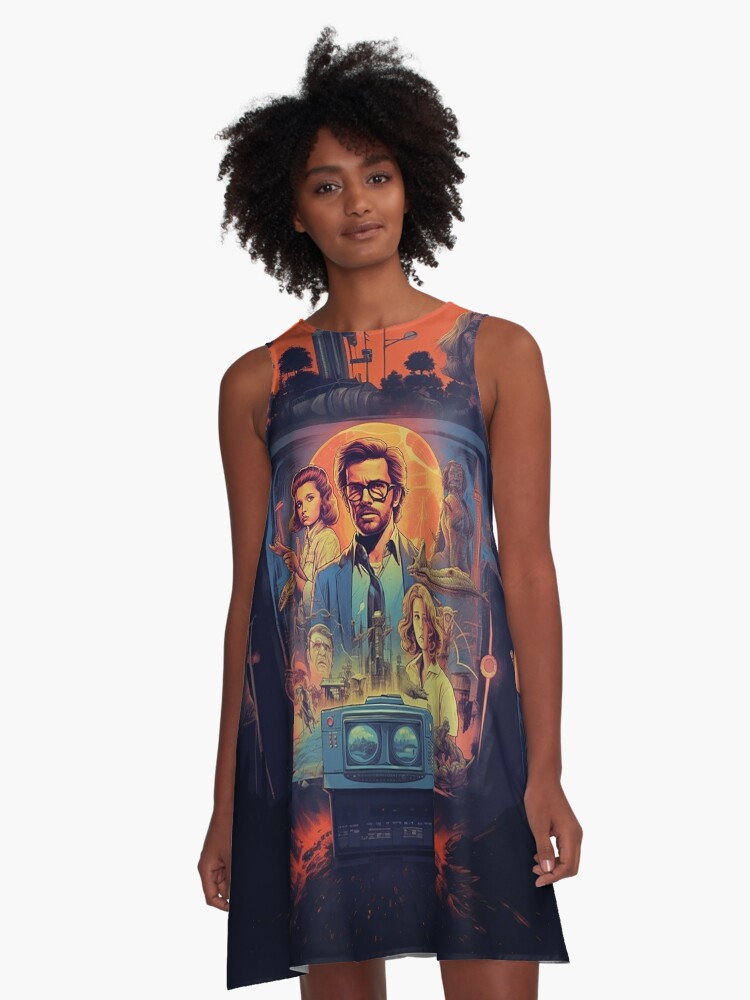A striking photograph features a young black woman standing confidently with her arms at her side, her medium-length, frizzy hair framing a gentle smile. She wears a graphic t-shirt dress that is both vivid and intricately detailed, resembling a retro sci-fi movie poster. The dress showcases an elaborate scene with various characters and elements. Dominating the center is a white man wearing glasses, a blue suit, and a blue tie, suggesting an intellectual or authoritative figure. Flanking him are multiple women: one with a mid-century haircut, another with curly blonde hair and a white shirt, and a third whose attire is indiscernible. Additionally, an older man and a robot are present among the characters. The backdrop of the scene includes a vivid orange skyline and machinery, creating an ambiance of mid-century science fiction. The lower part of the dress features darker hues and dynamic elements reminiscent of solar flares or volcanic activity, adding to the dramatic and immersive quality of the print. The model's direct gaze and slight head tilt, paired with the vibrant and complex artwork, create a captivating and visually rich portrayal.